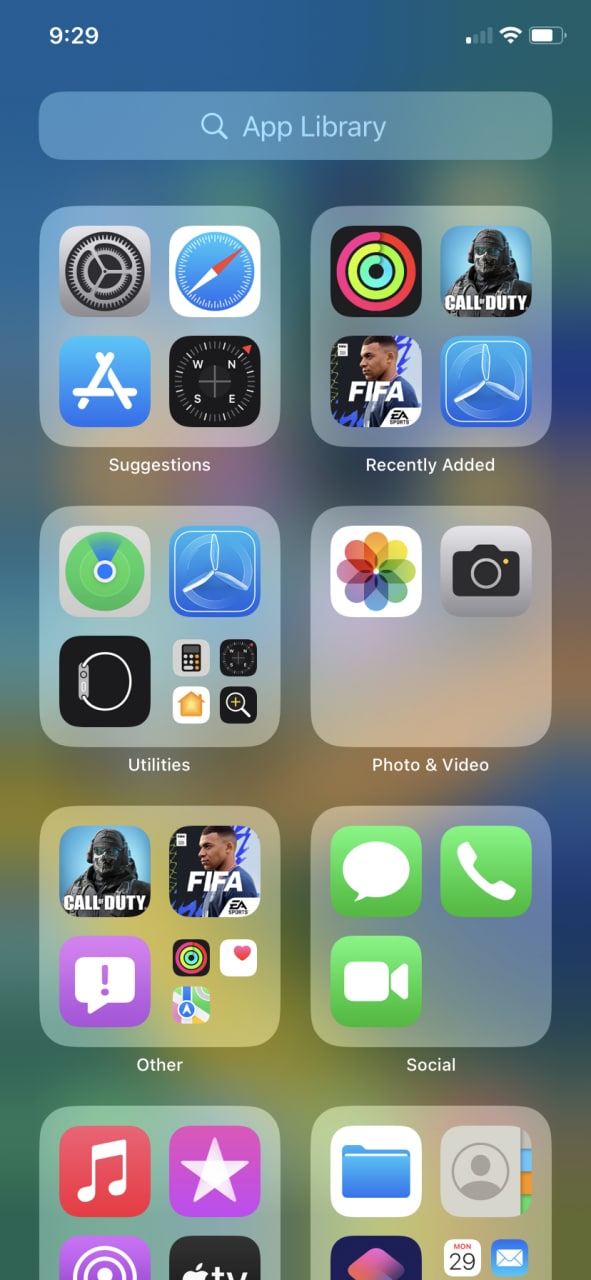Screenshot of someone's iPhone home screen featuring the default iPhone background. At the top, the status bar shows the time as 9:29 AM on the left. On the right, the signal strength is at one bar, Wi-Fi signal is full, and the battery is at three-quarters.

In the center, there's a light blue rectangle with a magnifying glass icon labeled "App Library." Below, the screen displays 8 app folders (4 in each row):

**Top Row:**
1. **Suggestions:** Contains icons for the Settings app, Safari browser, App Store, and the Compass app.
2. **Recently Added:** Includes a colorful bullseye icon, a Call of Duty game icon featuring a character from the game.
   
**Second Row:**
3. **FIFA:** Displays a player, though the specific player isn't identified.
4. **Adobe:** Shows a generic Adobe icon.
5. **Utilities:** Comprises a radar-like icon (app unknown), an Adobe icon, Apple Watch icon, and smaller icons for Calculator, Compass, the Home app, and Magnifier with a plus sign.
6. **Photos and Video:** Includes the Photos app icon (a multi-colored flower) and the Camera app. 

**Third Row:**
7. **Other:** Features a Call of Duty icon, FIFA icon, an unknown purple app with a white speech bubble and purple exclamation mark, and smaller icons including the bullseye from earlier, a white square with a red heart, and a map icon.
8. **Social:** Contains the Messages, Phone, and FaceTime icons.

**Partially Visible Folders:**
1. A red square with a white piano note.
2. A purple square with a white star.
3. Apple TV icon.
4. A white square with a blue folder.
5. The Contacts app.

Some folder contents and icons on the rightmost side of the screen are cut off and not clearly visible.